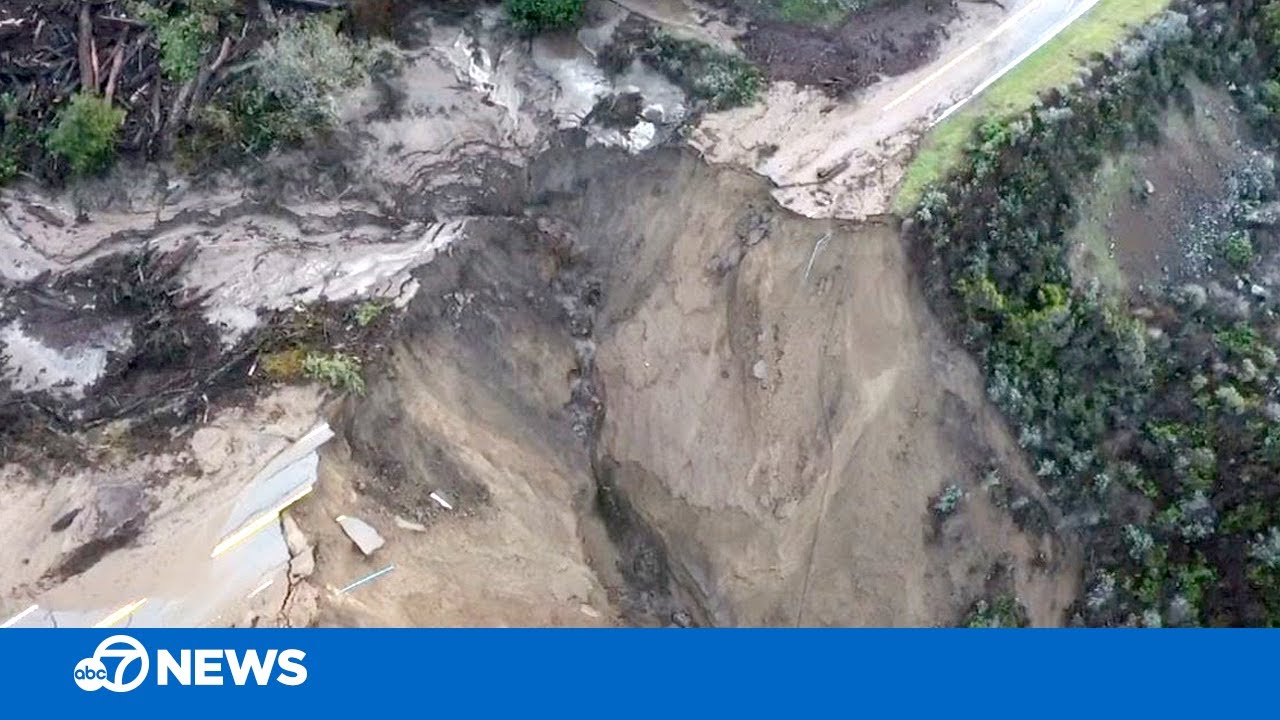The image captures an aerial view of a mountainside in daylight, likely a screenshot from a TV news broadcast. The striking scene centers on a massive landslide or mudslide that has severely damaged a road, splitting it with a jagged crevice and revealing both gravel and asphalt falling away at the edges. Dark, murky mud is seen oozing down the hillside into the crevice. On the bottom of the image, a blue news ticker reads "ABC 7 News" in white text. Surrounding the affected area, the landscape shows a mixture of green trees, some of which appear damaged, scattered on both the bottom right and top left of the photo.